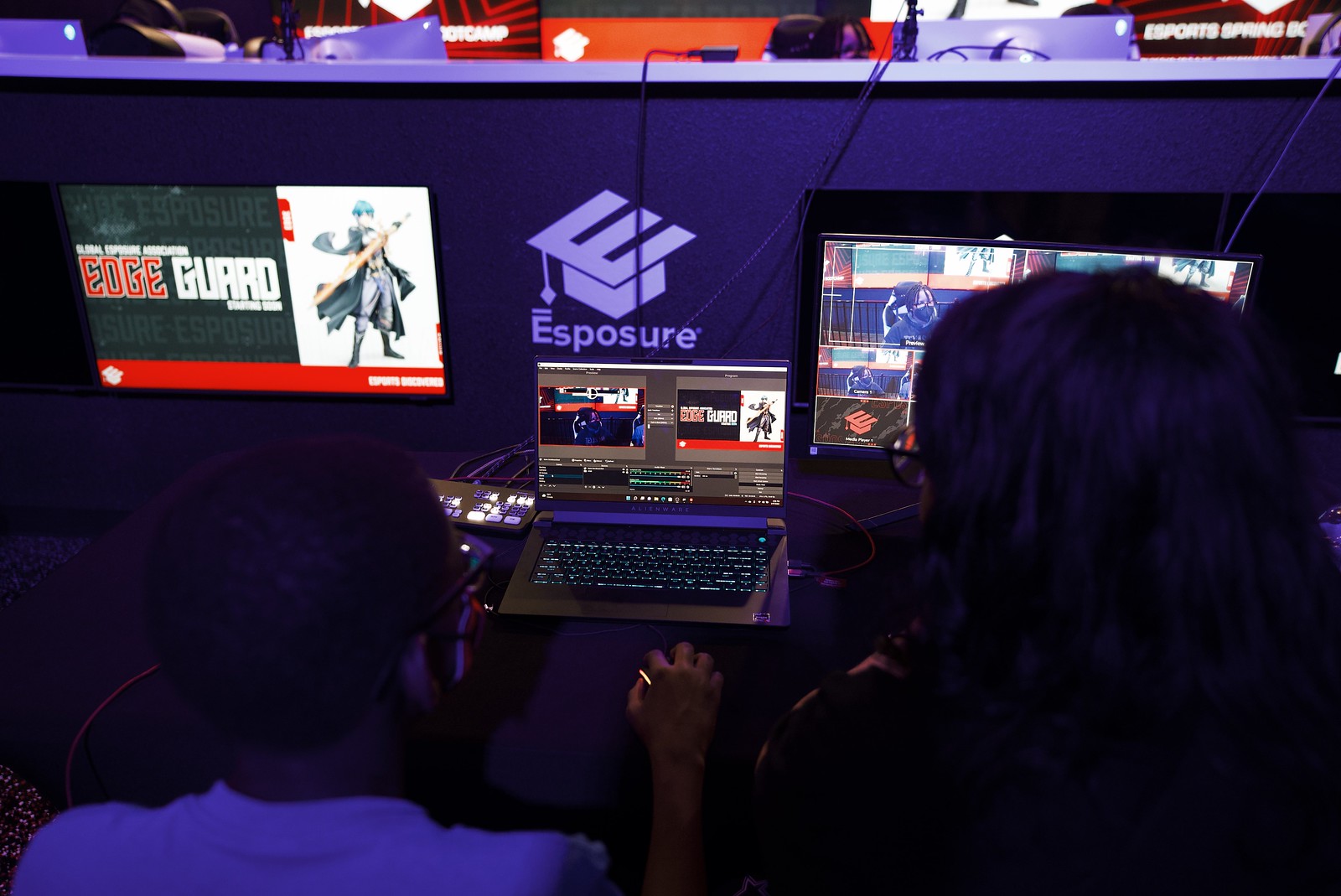The photograph captures an intense gaming atmosphere at what appears to be a gaming cafe or esports event. Two individuals are seated in front of a setup comprising three monitors. Positioned on the left is a TV displaying the game screen titled "EDGEGUARD," with "EDGE" in bold red letters and "GUARD" in white, accompanied by a fantasy male character adorned in flowing robes. The center monitor is a laptop, while the right monitor is mounted on a stand. Behind the monitors, a purple wall proudly displays the white "ESPOSURE" logo, featuring a stylized graduation cap shaped like the letter "E." The individual on the left, a male wearing glasses, seems focused on controlling the mouse, while the individual on the right, likely a female due to her long hair and glasses, is equally engrossed. The scene is captured indoors, reflecting a competitive and collaborative environment.